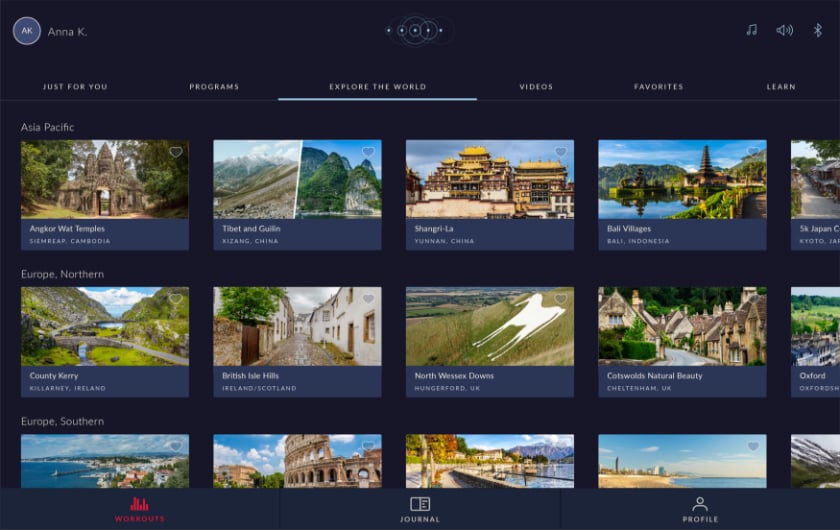A sleek black-themed website prominently features a minimalist design. In the upper left corner, there is a small blue circle with a white outline, containing the initials “AK” in white at the center. Adjacent to this icon, the name "Anna K" is displayed in white text, with "Anna" spelled with two Ns. Central to the interface are five white dots arranged horizontally, acting as a navigation aid.

On the right side of the screen, there are icons representing Bluetooth, sound settings, and music options. Beneath these icons, a horizontal navigation bar presents several links: "Just For You," "Programs," "Explore The World," "Videos," "Favorites," and "Learn."

The main content area is organized into three rows of images. Each row contains five images, though the fifth image in each row is partially cut off. Specifically, in the top row, the first image is identified as the Angkor Wat Temple in Siem Reap, Cambodia. The subsequent images depict locations in Tibet, Guilin in Guangxi Province, China (though noted with a typographical error as "K-I-Z-A-N-G"), and Shangri-La in Yunnan, China. The last image in the row is partially cut off and unidentified. The bottom two rows share a similar cutting-off pattern on both the bottom and right segments, highlighting the ongoing visual theme of partially hidden content.